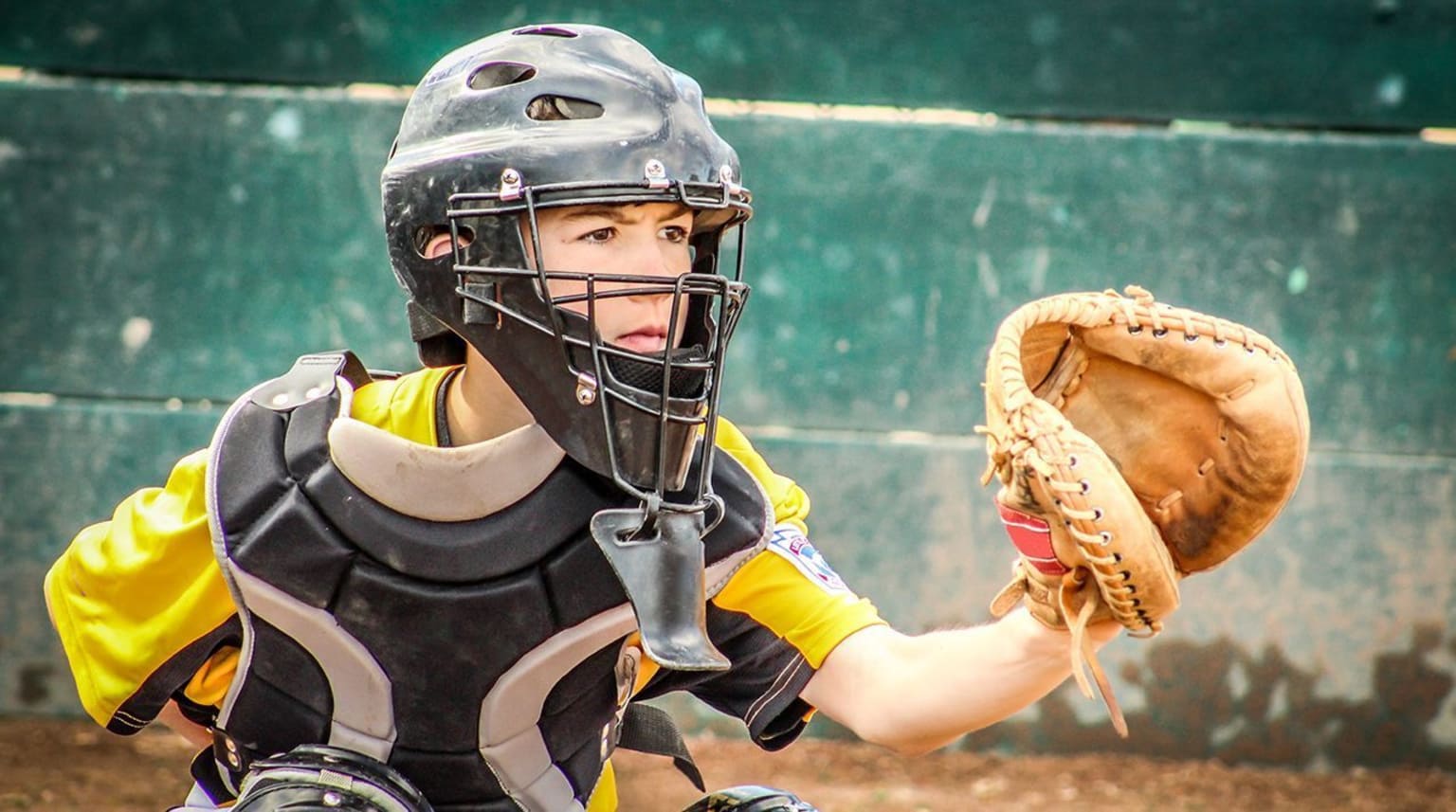A full-color photograph, taken outdoors in natural light, captures a young boy, approximately 10 to 12 years old, positioned as a catcher in a baseball game. The image is horizontally rectangular with no border, and the background features an aged green wall composed of three vertical panels, marked by white lines. At the bottom of the frame is a patch of brown dirt from the field.

The boy is crouched down in a ready stance, looking intently towards the action. He wears a heavy-duty black helmet with a protective face grid, complete with a neck guard. His uniform consists of a yellow and black jersey, covered by a black and gray chest protector that extends across his shoulders and chest. In his left hand, which is positioned up and out to his right due to the crouch, he holds a large, light brown leather catcher's mitt. His right hand is bent and tucked behind his back. The overall composition suggests the boy is focused and prepared, embodying the essence of a young catcher in the midst of a game.